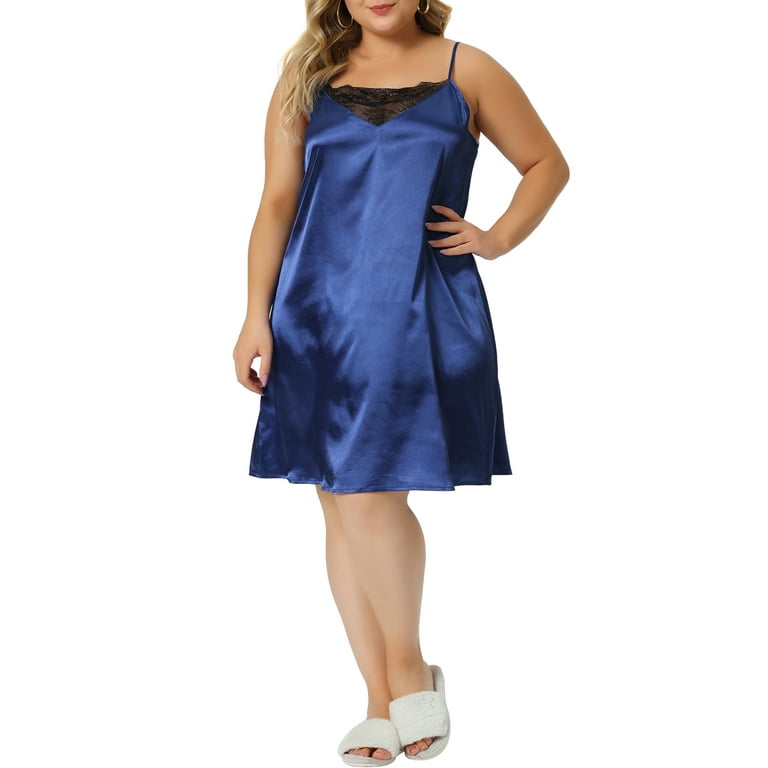The image features a Caucasian woman with wavy, ruddier blonde hair, and hoop earrings, wearing a velvety, satiny slip-on dress in a dark, royal blue color with black lace details. Her face is cropped out just above the lips, showing her red lipstick and a slight smile. She stands in a white void, suggesting a photoshopped background likely intended for advertising or a catalog. Her stance has her legs close together, her right arm relaxed by her side, and her left hand resting on her hip. She is also wearing fuzzy, off-white slippers, giving the appearance of an outfit intended for sleepwear or loungewear.